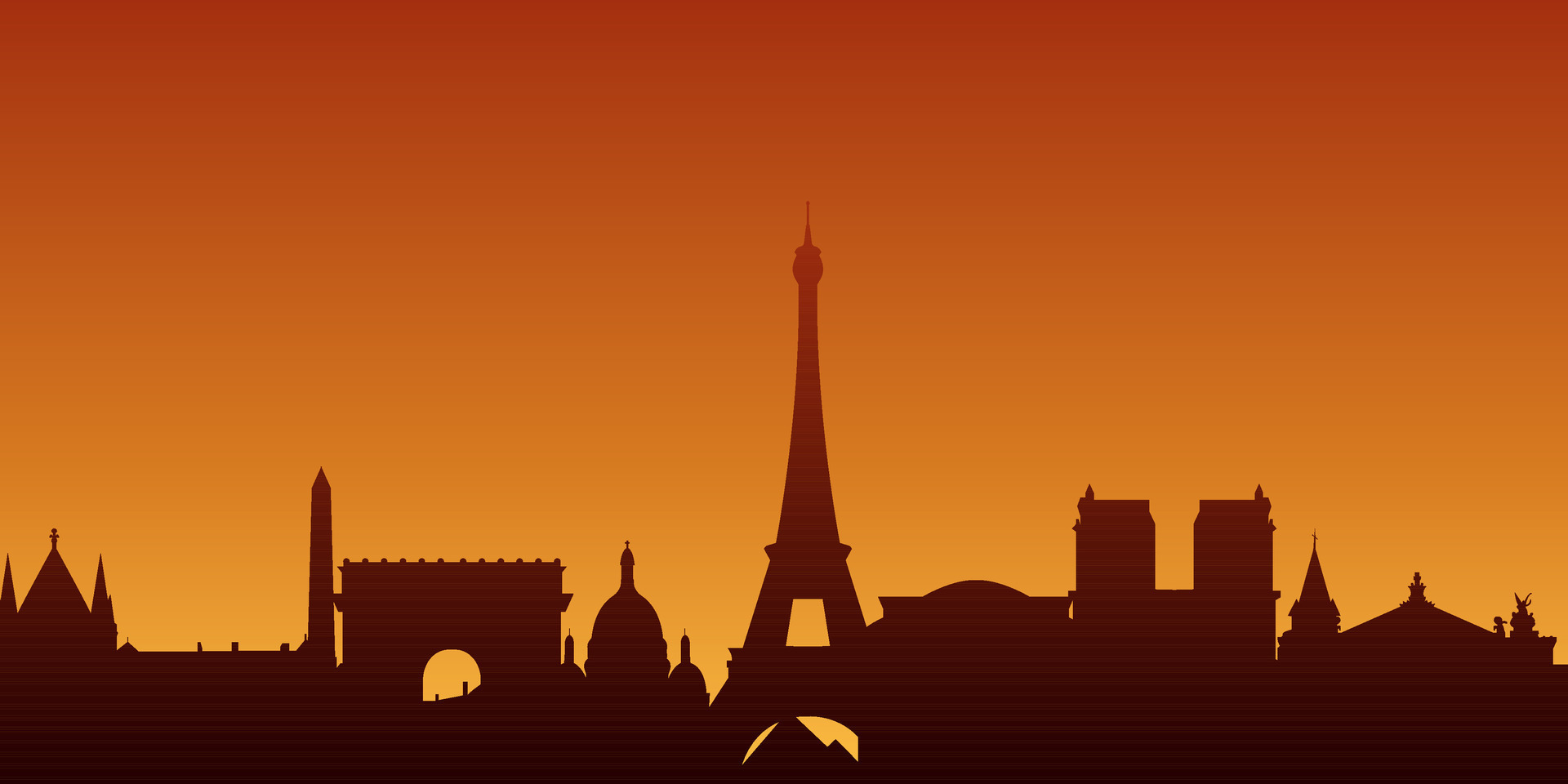This image is a computer-generated, animated silhouette of the Paris skyline during sunset. The background features a gradient of warm hues, transitioning from a lighter orange at the bottom to a darker, almost reddish-orange at the top. The central focus of the skyline is a distinctly A-shaped Eiffel Tower, which stands taller than the other structures. Surrounding the Eiffel Tower are various iconic Parisian landmarks, including the Arc de Triomphe situated to its left, and an array of churches marked by their steeples and domes. The buildings are tightly packed together, more so than in reality, suggesting an artistic montage of France’s most recognizable monuments. The entire scene is rendered in black silhouettes against the vibrant sunset sky, creating a stark contrast and emphasizing the iconic shapes of the city's architecture.